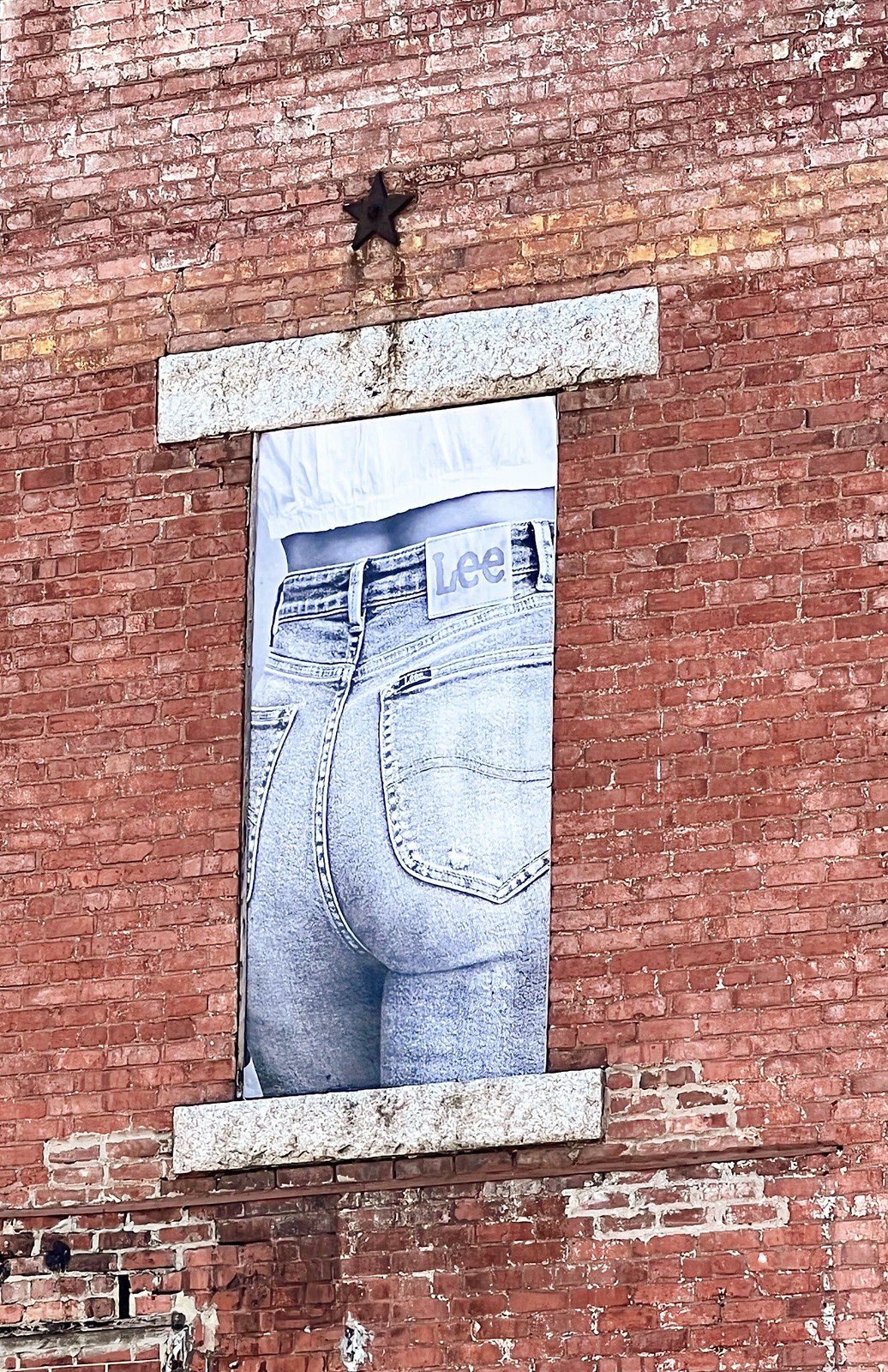This image features a close-up view of a person wearing jeans, focusing on the waist to upper thigh area, emphasizing the rear pocket and contours of the buttocks prominently. The background presents a multi-colored brick wall, with an intriguing gradient effect: the top rows of bricks are more white than orange, transitioning to predominantly orange bricks in the center, and then to a mix of orange, white, and black bricks at the bottom. Set into the wall is a window-like structure framed by granite slabs on the top and bottom. This feature does not contain glass but rather displays a picture. Above this pseudo-window, a black star icon commands attention. The overall composition juxtaposes the detailed textures and color variations of the brick with the fabric and form of the jeans-clad figure, creating a visually intriguing scene.